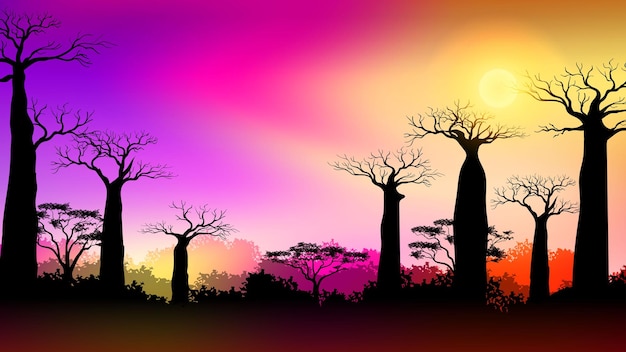The image is a highly stylized and vibrant illustration, not a photograph, depicting a striking landscape. The rectangular frame, longer than it is tall, captures a dramatic sky transitioning through various tones of purple, magenta, and yellow. On the right side, a faint sun peeks through the haze, casting a yellow tinge that fades into magenta, pastel lilac, and deep purple hues as it spreads across the sky. The horizon showcases a blend of pastel shades of purple, orange, and yellow, enhancing the visual contrast.

In the foreground, the silhouettes of diverse trees stand out starkly against the colorful backdrop. Barren trees with thick trunks and bare branches dominate the scene, interspersed with a few trees featuring slender branches and sparse leaves at their tops. A dense, dark silhouette of shrubbery and foliage occupies the lower part of the frame, contributing to the overall shadowy foreground.

The image's aesthetic might evoke an African savannah with its characteristic trees, though rendered in a cartoonish or animated style. The combination of vibrant sky colors and black silhouettes gives the illustration a surreal, artificial look, highlighting the beauty of nature through an imaginative, graphic art lens. The sun setting or rising in the distance and the intricate play of colors create a captivating visual experience, balancing the vivid sky with the dark, grounded elements.